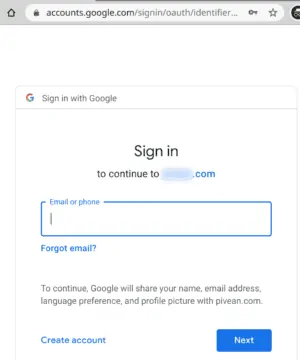The image showcases a Google sign-in page with various interactive elements and textual information. 

- **Top Right Corner:** There is a star icon.
- **Top Left Corner:** An upward-pointing arrow is visible. 
- **Address Bar:** Situated next to the arrow is a search or address bar. A padlock icon precedes the site address.
- **Main Body:**
  - **White Space:** Below the address bar is some white space.
  - **Google Logo:** The Google logo is prominently displayed.
  - **Sign-in Text:** The text reads, "Sign in with Google."
  - **Instructions:** Below it, a sentence instructs the user to "enlarge your print," followed by, "sign in. To continue to," but the following word is blurred.
  - **Text Box:** There is an empty text box with a blue border, labeled "Email or phone" in blue text. The cursor is positioned at the beginning of this text box. Below it, the blue text "Forgot email" appears.
  - **Privacy Notice:** The text explains that Google will share certain user information, including name, email address, language preference, and profile picture with pivian.com. This is written in dark gray or black text.
  - **Action Button:** A medium blue rectangle contains centered white text that reads "Next."
  - **Account Creation Link:** To the left side, "Create account" is written in blue text against the white background.
- **Footer:** The rest of the page is blank, except for the Google 'G' logo at the top.

There are no additional photographs or logos present on this page.